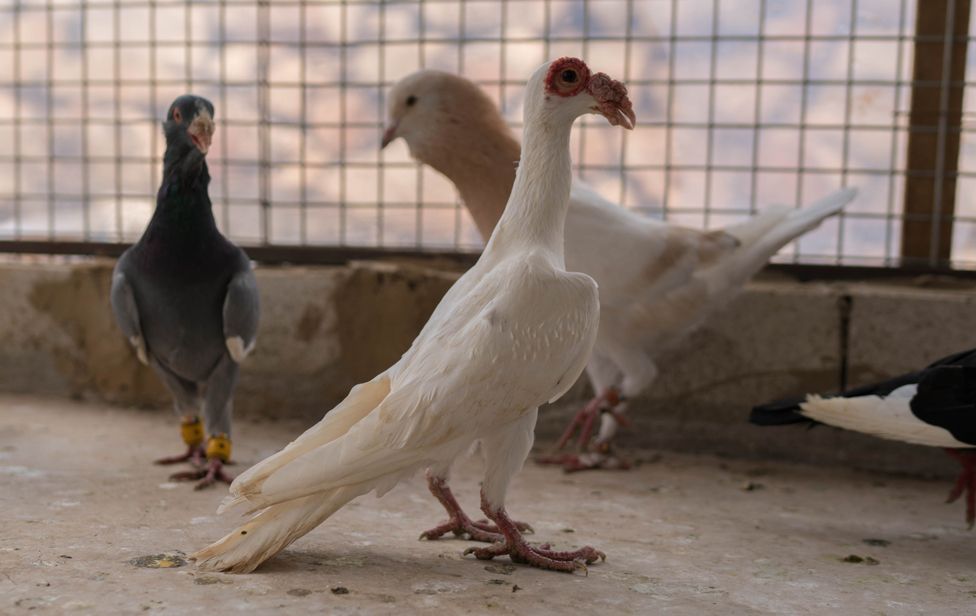In the image, three distinct birds are confined within an enclosure featuring a dirty, dusty concrete flooring and a wooden gate with a checkerboard wire mesh at the top. The bird at the center stands out with its slender white body, black eyes, and a unique, bumpy beak adorned with red patches. This bird also has dark orange, wrinkled feet equipped with small talons. Behind it is another white bird, characterized by a much fluffier face and a notably larger overall appearance compared to the central bird. To the right, the tail feathers of a predominantly black bird are visible; these feathers showcase long whitish tips. On the left, there is a grayish bird with distinctive white tips on its wings and orange rings around its claws. The birds' positioning and the dilapidated state of their surroundings hint at captivity.